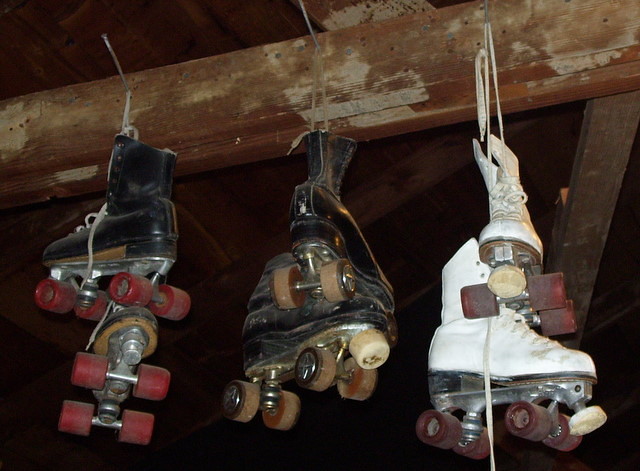In this photograph, taken in what appears to be a dimly lit basement, there are three pairs of vintage roller skates hanging securely from large, angled nails hammered into a sturdy wooden beam. The skates are suspended by their well-worn laces, which are looped around the nails to keep them in place. The background features old, dark brown rafters with patches of faded white paint, further suggesting the age and rustic nature of the setting.

The skates, which have noticeably wide ankle material for lacing, exhibit signs of significant wear and age. On the left hangs a pair of black roller skates with vibrant red wheels. In the middle, another pair of black skates is distinguished by its dark brown wheels, likely faded from their original color. The pair on the right stands out with its white boots and matching red wheels. Despite their aged appearance, the skates hang sturdily, indicating that they have been preserved for many years. The different sizes of the skates hint at usage by various individuals, though it's unclear whether they were meant for children or adults. The overall scene evokes a sense of nostalgia, capturing a simple yet vivid snapshot of the past.